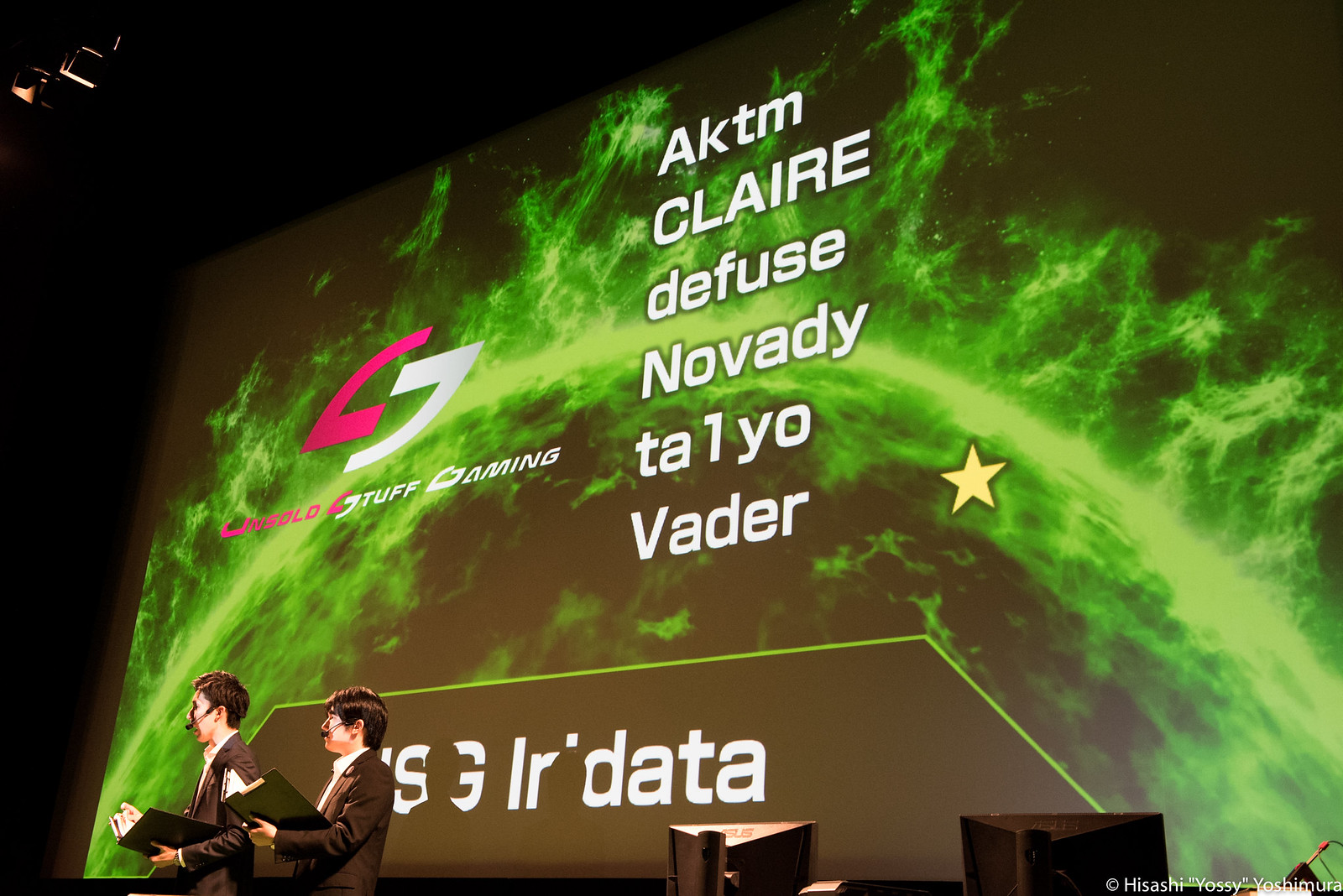The image captures two men in black suits with white collared shirts, each equipped with ear microphones and holding portfolios with black covers, standing on a stage at an esports event. Behind them, a large banner features the names "AKTM, Claire, Diffuse, Novity, Ta1Yo, Vader" in white font. The banner is brightly illuminated by spotlights visible in the upper left corner of the image. Below the banner, there is a stylized image resembling a sun with green solar flares, accompanied by the text "Unsold Stuff Gaming". The stage setup includes a table with two black computer monitors. Above the text, there's a distinctive "G" symbol formed by two characters, one flipped 180 degrees. The camera angle, pointed slightly upward, captures the grandeur of the stage, emphasizing the scale of the event.